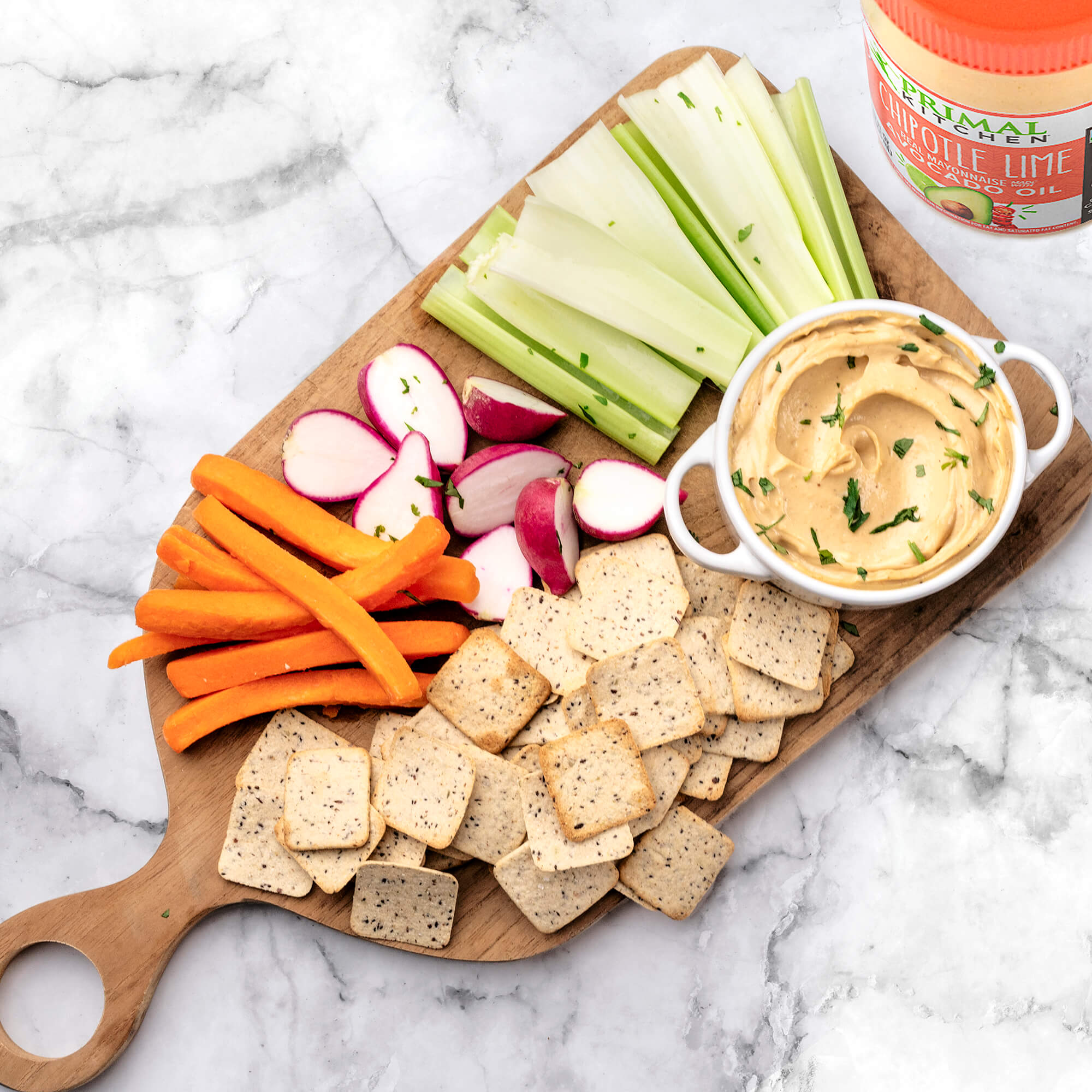The image depicts a detailed arrangement of a vegetable and dip charcuterie board placed on a marble or quartz countertop. The board itself is wooden, rectangular, and features a handle with a circular hole for easy handling. On this board, a variety of items are meticulously arranged: 

- **Crackers**: Found near the bottom left; these square crackers contain green specks.
- **Carrots**: Positioned above the crackers to the left, these are peeled and sliced into thin, finger-like shapes.
- **Radishes**: Centrally located next to the carrots, cut in half to reveal their red exterior and white interior.
- **Celery**: Located in the top right corner, cleaned and cut into sticks.
- **Dip**: In the bottom right, a white ramekin-style bowl with two small handles holds a creamy dip that has a peach hue, garnished with sprigs of parsley. This dip is identified as Chipotle Lime Avocado Oil Mayonnaise, given the presence of a labeled bottle to the right of the bowl.

The entire composition is accentuated with additional parsley sprigs scattered across the vegetables and dip, adding a touch of green.